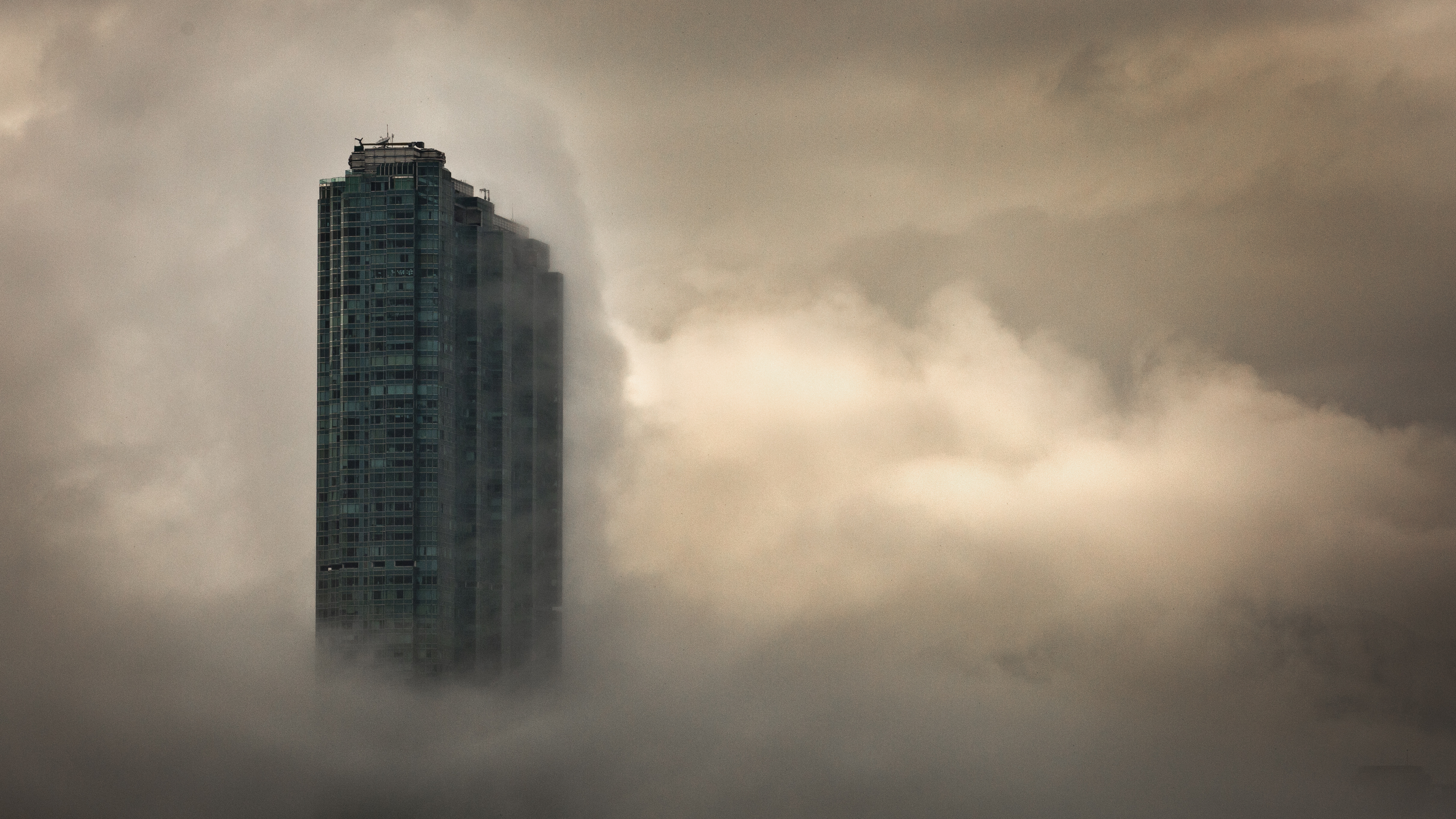In the photograph, a singular building emerges majestically from a sea of thick clouds. The image is taken from a considerable distance, which renders it as the sole structure visible amidst the cloud cover. The building itself is enveloped by white clouds that drift around its edges, occasionally shrouding parts of it and imparting a mysterious aura. The play of light and the misty veil make it challenging to discern specific details, creating an illusion that some windows might be missing. However, upon closer inspection, it appears that it's probably just the perspective influenced by the clouds. Satellite dishes are perched on its top, emphasizing its modern functionality. The building predominantly exhibits a bluish hue, likely reflected by the windows that remain clear of the clouds' embrace. The sky above is not the traditional blue but rather a foreboding gray, suggesting the presence of a dust storm or dense fog, adding an eerie atmosphere to the scene.